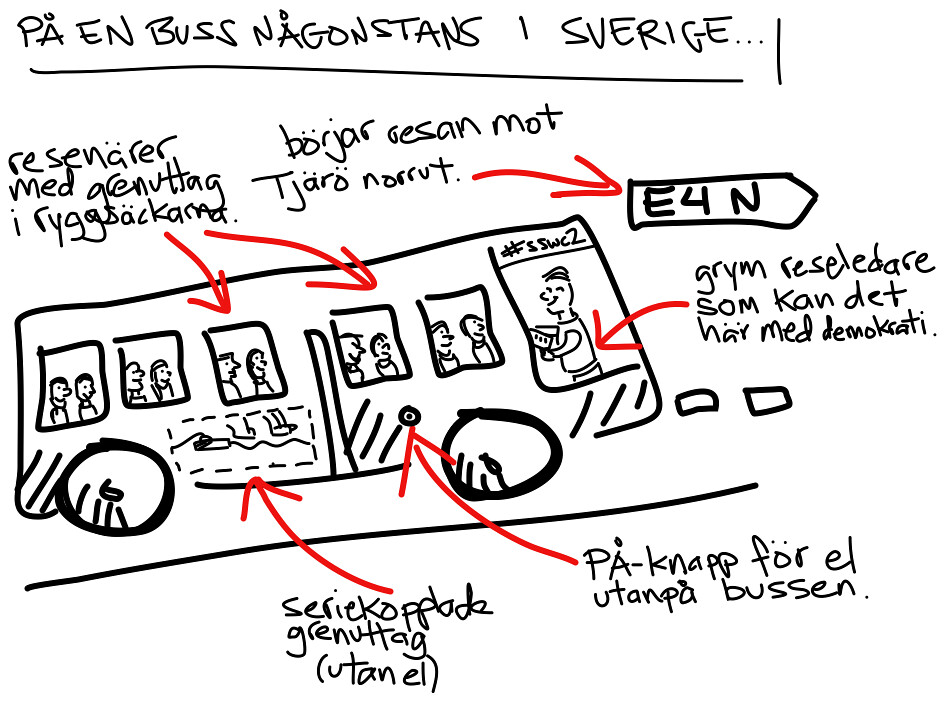This detailed black ink drawing, potentially rendered digitally, depicts a bus accompanied by text in a foreign language. The bus serves as the focal point of the artwork, which includes multiple red arrows pointing to various parts, likely identifying different components. Significant text at the top suggests a title, rendered as "Pa-N-Bus Nagonstansfergy," with an additional arrow pointing inside that reads "E4N." The bus features five windows, each populated by two passengers, totaling ten seated individuals, identifiable by attributes such as short or long hair. At the front, a standing figure likely represents the driver. In front of the bus are two small squares, possibly signifying the road or surrounding environment. Transparent, dotted rectangles at the bottom suggest a view of the passengers' legs, giving a layered perspective. The image uses black ink predominantly, with red as the only contrasting color employed for the arrows and text.